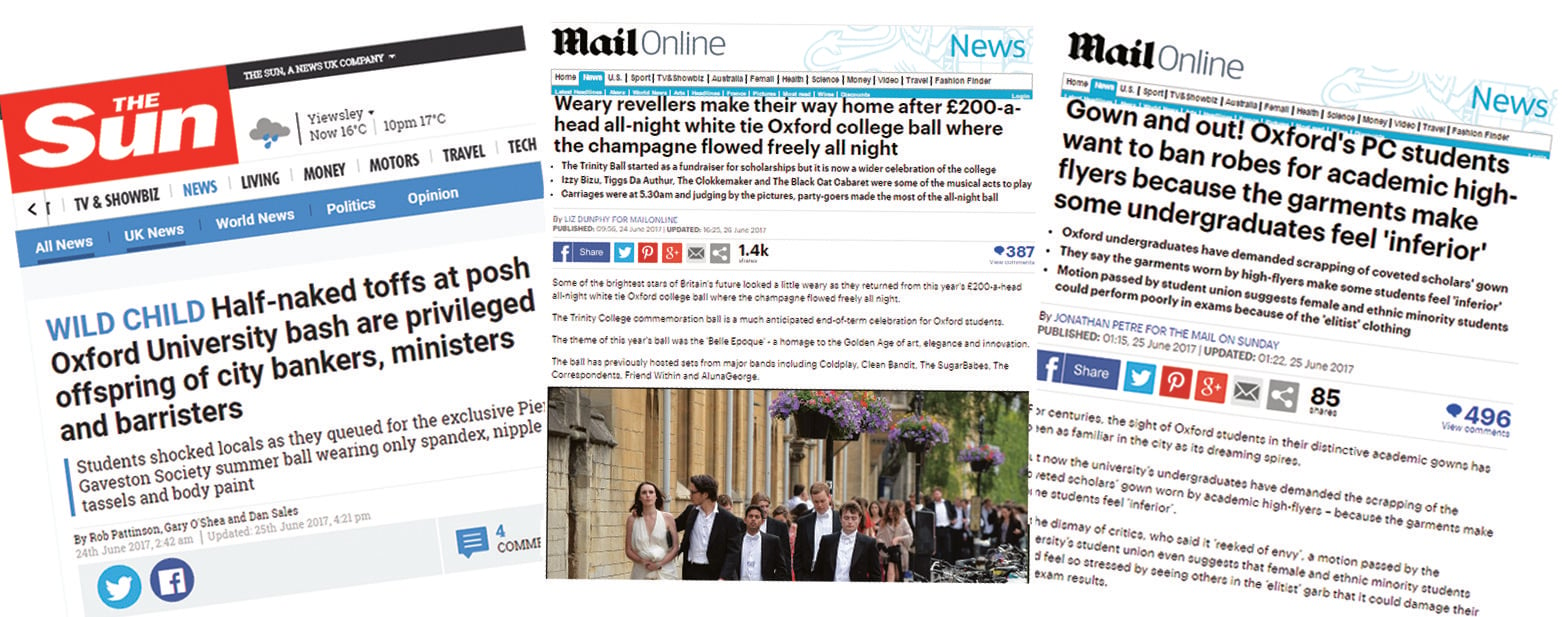**Caption:**

In a juxtaposed display of tabloid and online media coverage, three images of articles from The Sun and Mail Online are aligned side by side. 

The leftmost image captures an article from The Sun, which is slightly tilted to the left. Dominated by its iconic red box logo in the upper left corner inscribed with "The Sun" in bold white letters, the article begins with a vivid headline: "Wild Child." These words are highlighted in blue, contrasting with the remaining black print. The headline reads: "Wild Child: Half-naked toffs at posh Oxford University bash are privileged offspring of city bankers, ministers, and barristers." Beneath this, a subtitle in black text provides additional context, followed by the author's name, the article's date of publication, and social media icons for Facebook and Twitter (now rebranded as X). Adjacent to the logo is a daily weather report and a navigational menu featuring options such as 'TV & Showbiz,' 'News' (selected), 'Living,' 'Money,' 'Motors,' 'Travel,' and 'Tech.'

The central image focuses on an article from Mail Online, presented in a straight, vertical orientation. The headline, printed in black, declares: "Weary revelers make their way home after 200-pound-a-head all-night white-tie Oxford College ball where the champagne flowed freely all night." This is supported by three subtitles, which are followed by social media icons for Facebook, Twitter, Pinterest, Google+, and an email sharing option. Below the text, a photograph portrays a group of college students dressed in tuxedos and gowns, making their way home in the early morning light.

To the right, an article from The Sun mirrors the first but is inclined slightly to the right, completing this triad of media reportage.